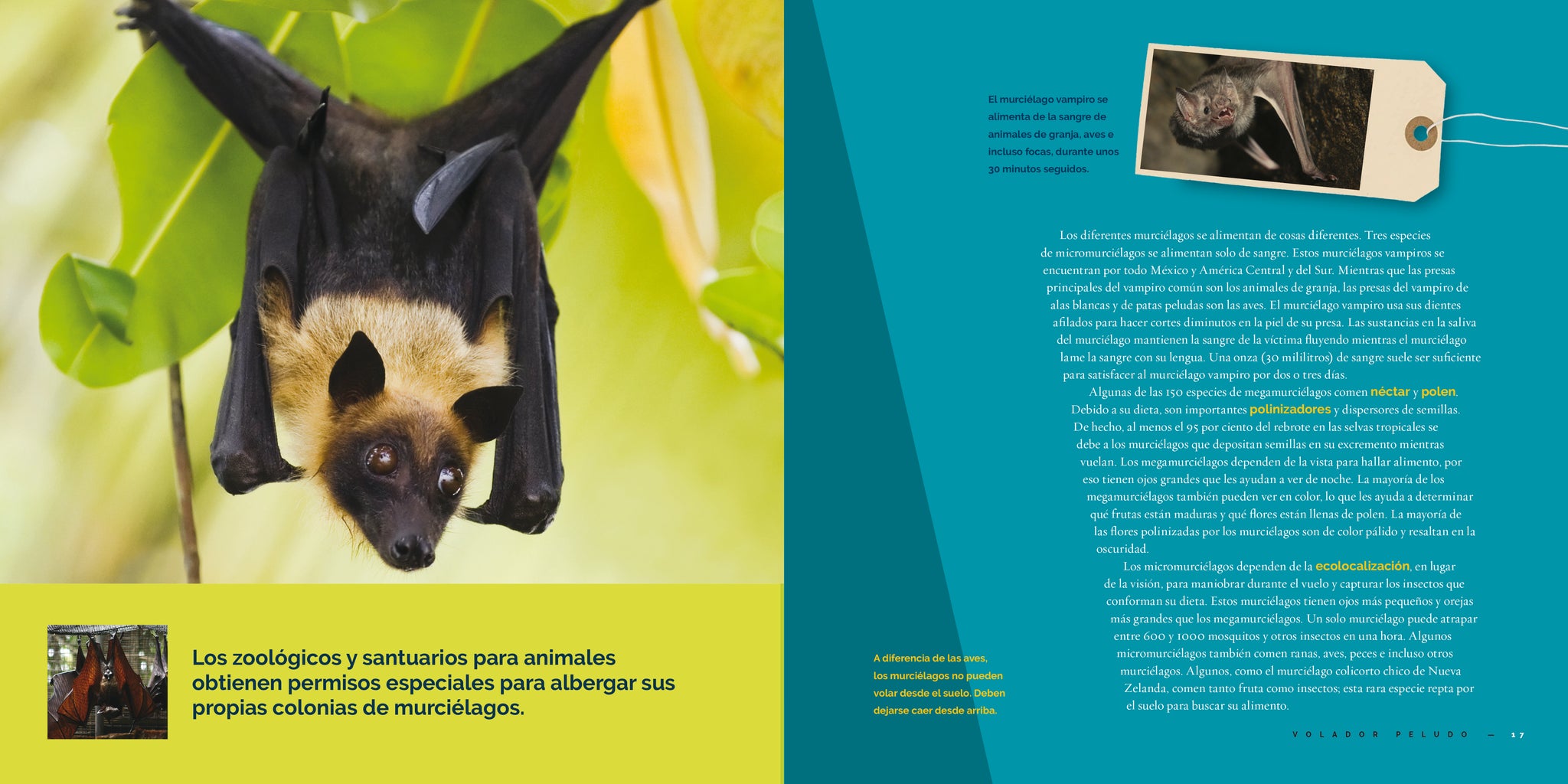The image is a detailed poster or pamphlet in Spanish about bats. On the left side, there is a close-up image of a bat hanging upside down from a branch amidst green and yellow leaves. The bat has a gray and light brown fur with beige stripes and dark ears, its wings folded. Its eyes are open and brown, giving it a cute appearance, suggesting it might be a fruit bat. The background is slightly out of focus with lime green and gray hues, enhancing the vibrant foliage around the bat.

On the right side, a smaller image of a bat attached to a label with a string is displayed. This side features a light blue background with most text in white and some words highlighted in yellow-green and yellow text in the lower part. There's also some black text too small to read. The bat depicted here has a more menacing appearance, possibly indicating vampire bats, with noticeable teeth. The overall aesthetic includes colors such as green, gray, yellow, white, black, and blue, enhancing the informational and visual contrast between the two pages.